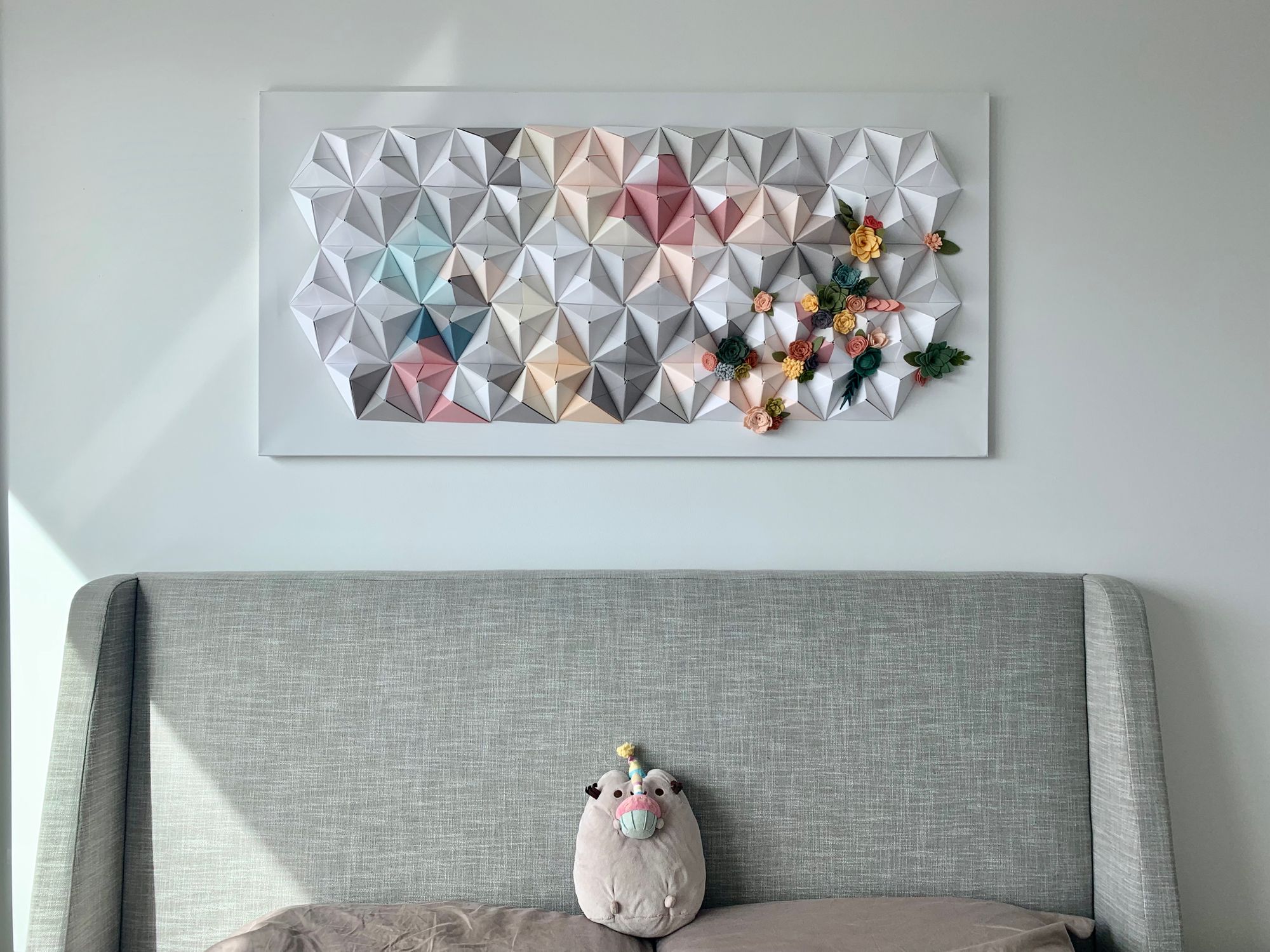The photograph captures the interior of a sunlit bedroom, predominantly featuring a gray headboard positioned centrally towards the bottom of the image. The bed is adorned with two dark grey pillows, and nestled between them is a gray stuffed toy resembling a sheep, whimsically holding a pink cupcake. Above the headboard, a striking rectangular artwork is mounted on the wall, characterized by its three-dimensional abstract geometric shapes, which are floral and cube-like in nature. The artwork's colors include shades of grey with accents of red, blue, pale yellow, and pink, and it adds a dynamic element with its textured, protruding pieces. To the right side of the room, there are yellow floral decorations further enhancing the serene yet vibrant ambiance. The wall behind the headboard is a calming shade of grey, creating a cohesive backdrop for the room's decor. Sunlight gently filters into the space, illuminating the thoughtfully arranged elements of this cozy, tranquil bedroom.